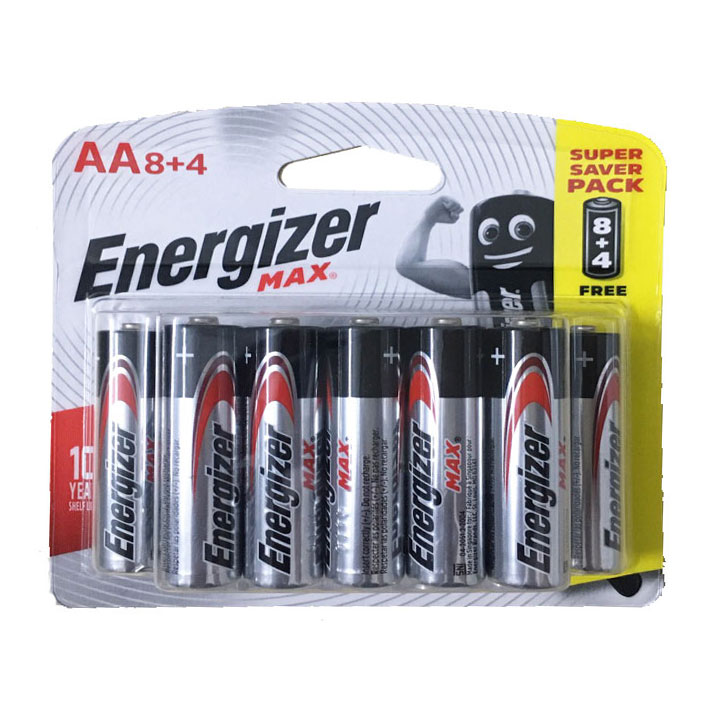This image depicts a close-up of a pack of AA Energizer Max batteries, isolated on a white background. The packaging is a blister pack with a cardboard backing featuring a shiny design, covered by a clear plastic overlay that securely holds the batteries in place. The batteries are displayed upright within their plastic casing.

Prominently displayed on the packaging is the Energizer logo along with the brand's mascot—an anthropomorphic battery characterized by cartoony eyes, a mouth, and a buff arm flexing towards the viewer. To the right-hand side of the packaging, a vertical yellow banner reads "Super Saver Pack 8," highlighting that the pack contains 12 batteries in total, including 4 free ones, as indicated by the "8 + 4 frees" message below an image of a battery.

On the left-hand side of the blister pack, there is a statement boasting a "10 years shelf life," suggesting that these batteries can retain their charge for up to a decade when stored properly. The image effectively emphasizes the branding, quantity, and longevity of the Energizer Max AA batteries.